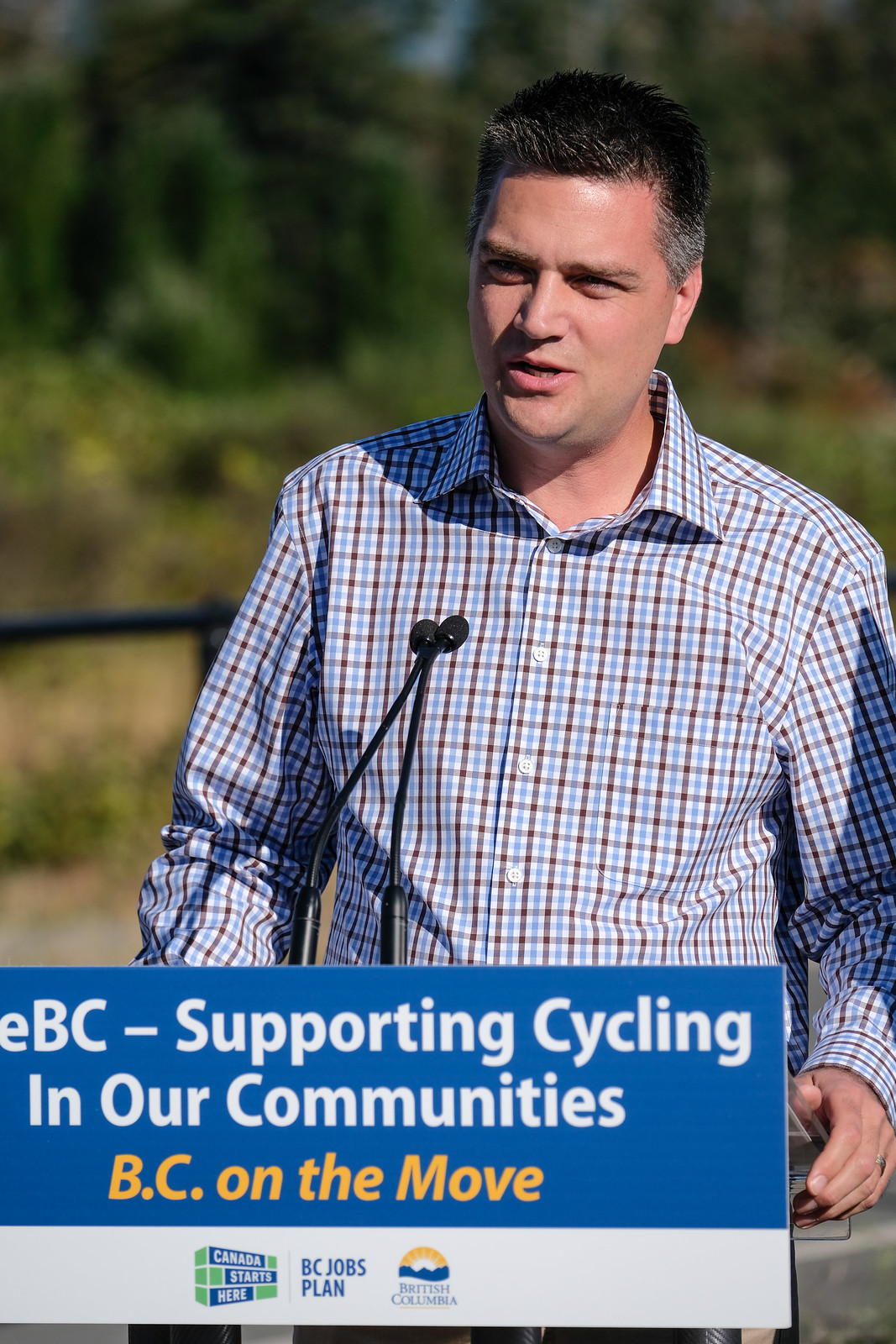This vertical image captures a middle-aged white male, appearing to be in his 40s, speaking into a thin microphone attached to a podium in an outdoor setting. The backdrop features a blurred array of trees and vegetation, indicative of a narrow depth of field and a photographer’s touch. The man, who has short cropped hair with hints of gray above the ears, is wearing a button-up plaid shirt in shades of white, blue, and brown. He stands confidently behind a blue and white podium adorned with a banner that reads, "EBC: Supporting Cycling in Our Communities" in white lettering, followed by "BC on the Move" in yellow, and additional text at the bottom stating, "Canada Starts Here - BC Jobs Plan." His left hand grips the side of the podium, displaying a silver wedding ring. The overall ambiance suggests a community event centered around cycling, possibly a race, emphasizing communal involvement and outdoor activities.